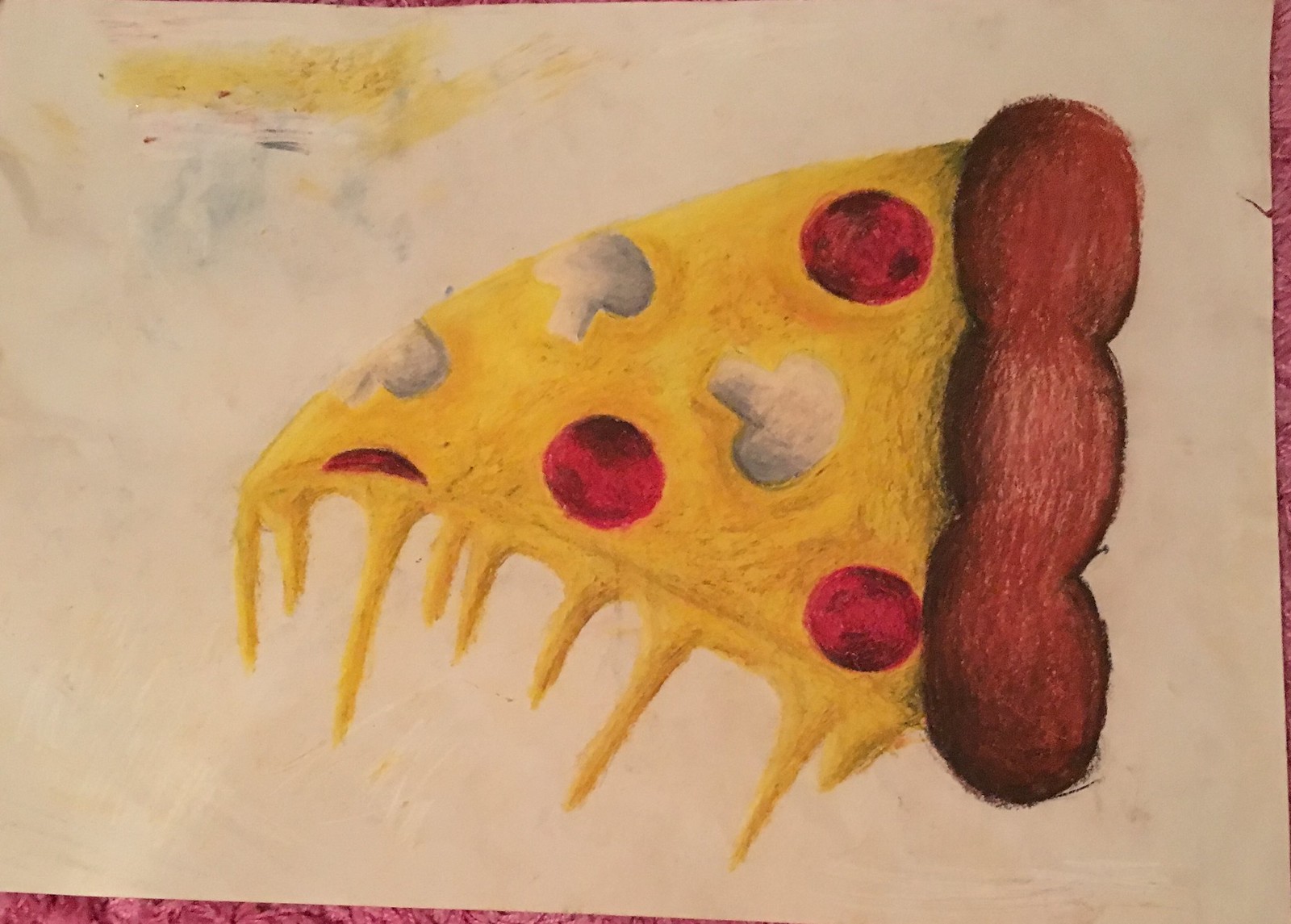This horizontal hand-drawn illustration, created with colored pencils or crayons, features a slice of pepperoni and mushroom pizza on a cream beige piece of paper, which has a slight rip on one side. The pizza slice is oriented sideways, with the pointed end to the left and the thick, somewhat puffy, reddish-brown crust to the right. The crust runs vertically and has undulating segments. The cheese, depicted in a bright yellow, drips severely off the lower edge of the slice in long, icicle-like projections. Three white mushrooms and three full slices of pepperoni, along with a sliver of pepperoni from where the slice has been cut, are scattered across the pizza. The illustration shows signs of previous attempts or smudges, with some yellow and green pencil markings in the background, possibly from testing colors or shading techniques. The paper rests on a brown surface, adding a touch of background context to the scene.